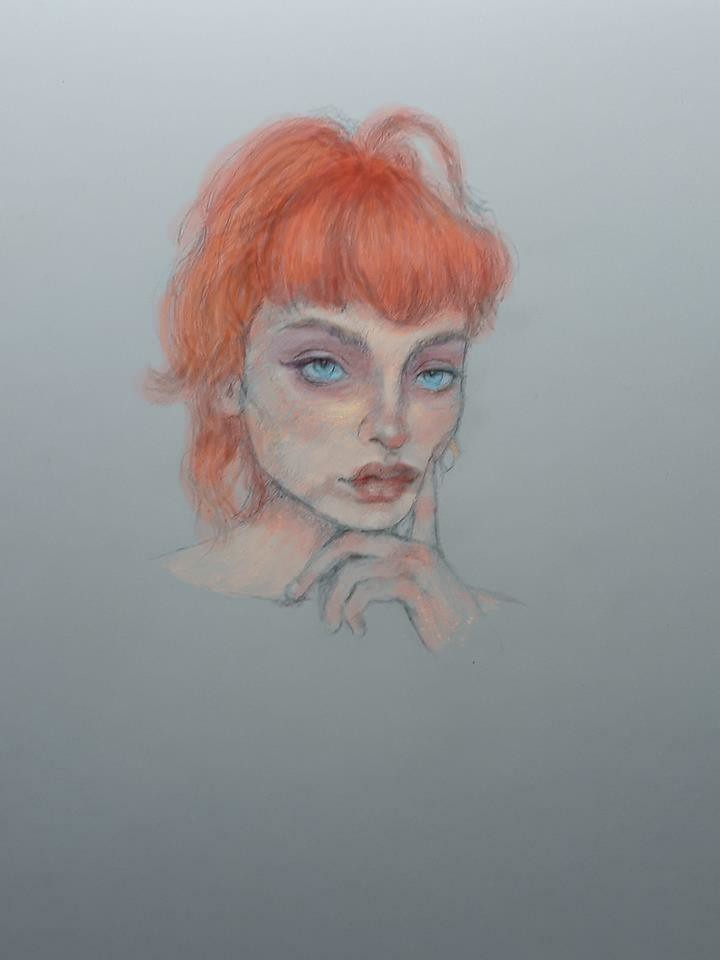The illustration is a detailed chalk or grease paint drawing of a red-headed woman with strawberry red, short hair that ends just above her shoulders. Her hair includes bangs that fall to the center of her forehead. She has fair skin with rose-tinted shading in areas that would traditionally have brown shading. Her blue eyes, framed by brown eyebrows and winged eyeliner, gaze directly at the viewer, though there is a distant, thoughtful expression in them, as if she is lost in contemplation. Her full lips are a darker shade of her hair color. She places her index finger of her left hand gently against her left cheek, causing a slight indentation, while the rest of her fingers are curled under her chin. The image captures her from the neck up, with her visible neck and no part of her body shown below that point. The drawing is set on light gray colored paper, and there is no artist's signature visible. The proportions of the image are taller than it is wide.